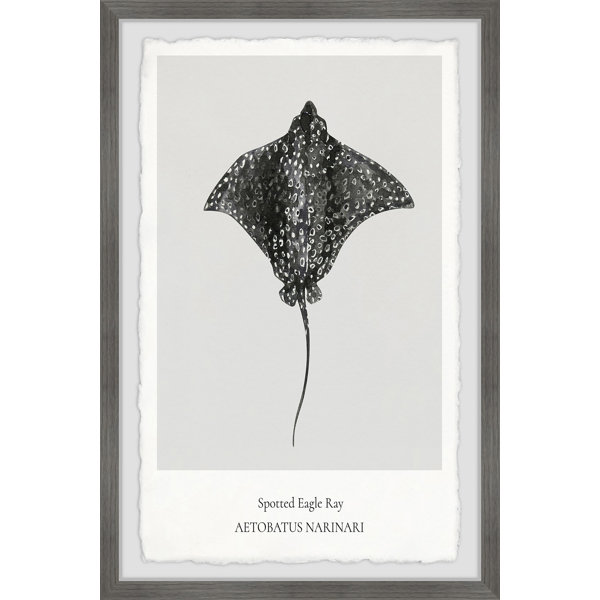This is a highly detailed framed black and white photograph of a spotted eagle ray (Aetobatus narinari). The frame is made of gray wood grain, adding a sophisticated touch. Inside the frame, there's a white mat border which provides a clean separation from the image. The photograph itself is placed within a further inner frame that appears almost like a tattered Polaroid, with thin white borders on three sides and a thicker white border at the bottom. This thicker bottom border bears the caption "Spotted Eagle Ray" in sentence case, and underneath it, in all caps, is the Latin name "Aetobatus narinari." 

The central image is a top-down view of the spotted eagle ray, which is oriented as if swimming upwards. Its broad wings are extended, and its long, thin, pointy tail trails elegantly behind. The creature is predominantly black, adorned with white spots arranged almost in a leopard-like pattern. The ray's small back fins are visible near the base of its tail, and it has a petite nose at the front. The meticulous details of the photo, along with the carefully crafted frame, make it a striking and informative depiction of this majestic marine animal.